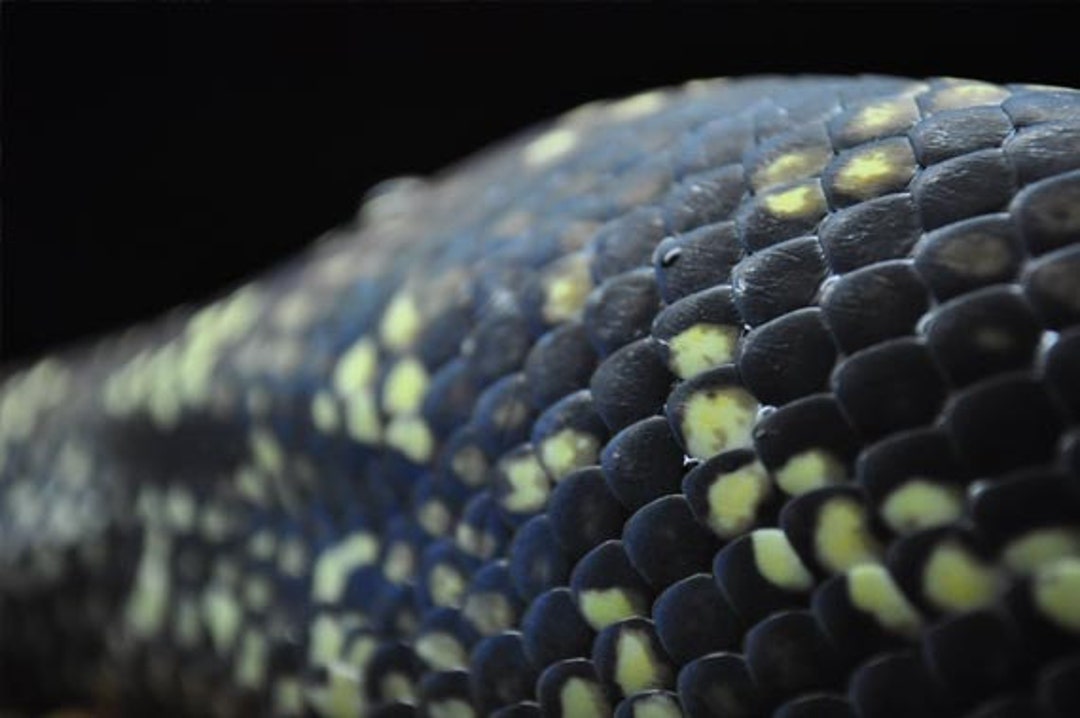The image is an extreme close-up of a reptilian or amphibian creature, likely a snake or lizard, captured in photorealistic detail. The scales, predominantly dark black, are hexagonal and appear pitched like tiles stacked atop each other. Interspersed among the black scales, there are dots and splatters of yellow and tan hues, which become more prominent towards the tail where additional brown tones can be seen. The background is pure black, possibly indicating that the image was taken in complete darkness or edited to remove any background distractions. Despite the high level of detail at the top of the image, the lower part blurs into the darkness, creating a gradient effect that contrasts the sharp details of the scales. The varied splashes of color and the segmented texture provide a vivid and intricate view of the creature's body.